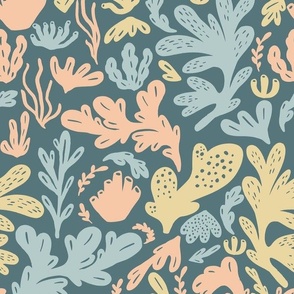This image features a print design that is likely intended as wrapping paper or decorative material. The design showcases an array of abstract, organic shapes that evoke the aesthetic of underwater flora and fauna. These shapes, which resemble leaves, seaweed, coral, and other marine growths, are rendered in a detailed, artistic style. The intricate shapes are reminiscent of paisley patterns and are distributed across a dark blue or gray background, which lends a deep, oceanic feel to the image. The palette comprises soft, pastel hues, including light blues, pinks, reds, and darker yellows, with each individual shape appearing in a single color. The overall effect is a harmonious and visually appealing composition that is suitable for gift wrapping for various occasions such as birthdays, weddings, or baby showers.